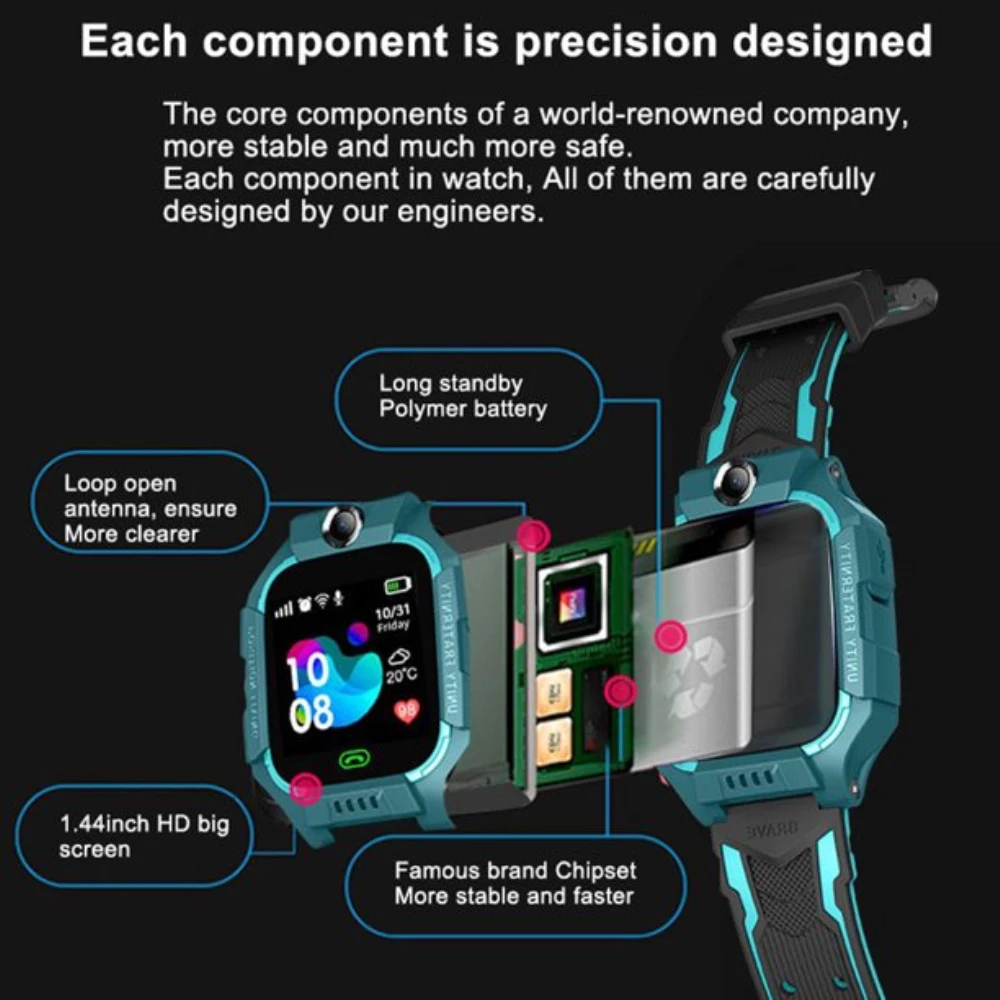This advertisement features a meticulously designed smartwatch, showcased in a turquoise and black color scheme, against a dark background. The image highlights the precision and craftsmanship of the watch, with detailed callouts for each component. These include a long-standby polymer battery, a loop-open antenna for clearer reception, a 1.44-inch HD big screen, and a renowned brand chipset that ensures stability and speed. The watch is presented disassembled layer by layer, illustrating the careful engineering by the company's designers. Text throughout emphasizes the precision design and superior quality of the core components, attributed to a world-renowned company, making the smartwatch both stable and safe.